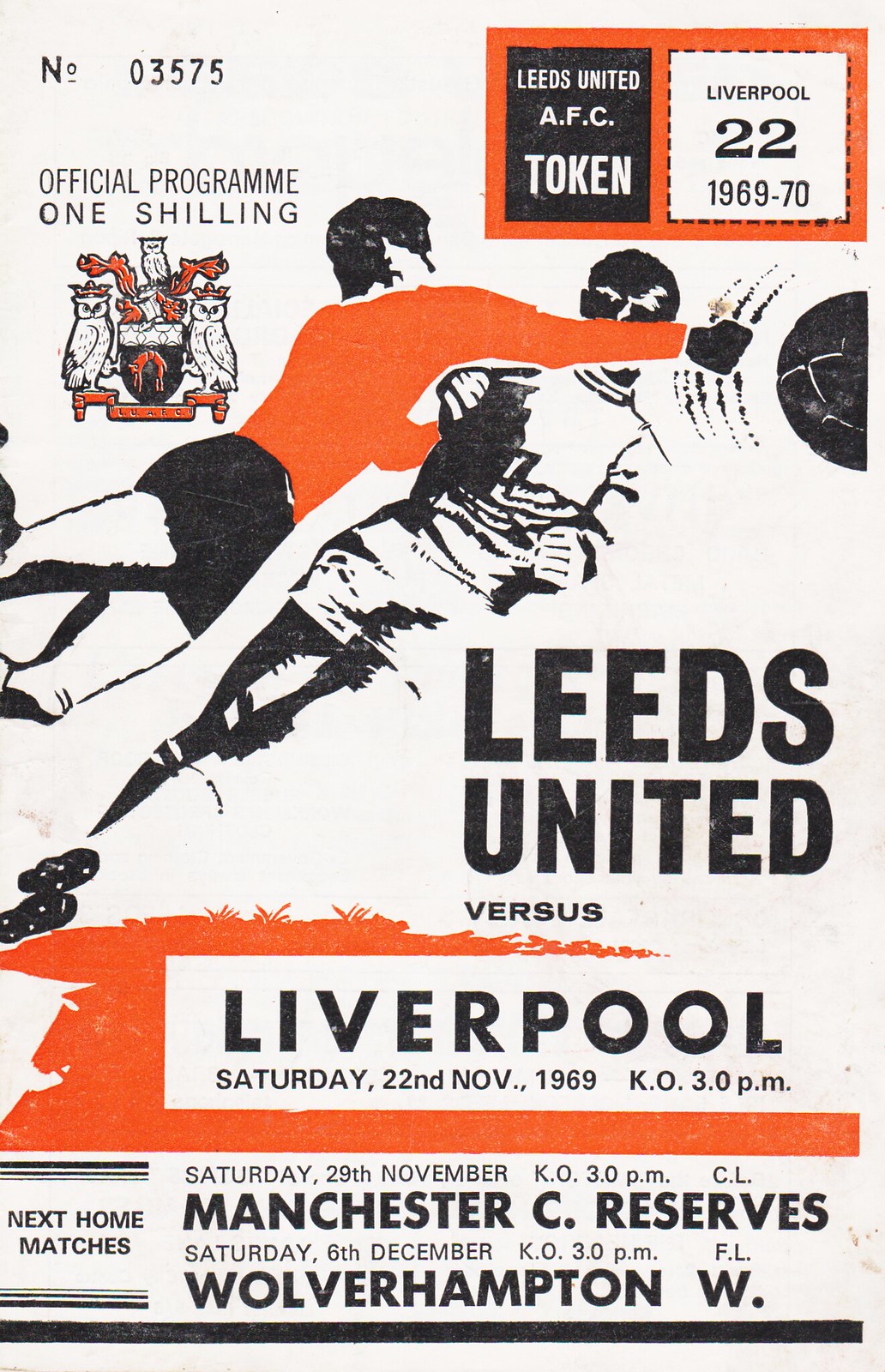The cover of the soccer program features a light gray background with black and orange print. At the top left, the program number "NO 03575" is prominently displayed, followed by the text "Official Program, One Shilling." To the right, it reads "Leeds United AFC Token, Liverpool 22 1969-70." Below this, two drawn soccer players are depicted in action: one in an orange jersey, possibly a goalie, leaping with another player beneath his arm, with the ball seen flying away in the scene. Midway down the page, the text "Leeds United versus Liverpool, Saturday 22nd November 1969, K.O. 3 p.m." is written in black font. At the bottom, a section announces upcoming home matches, listing "Saturday 29 November, K.O. 3 p.m., Manchester C. Reserves" and "Saturday 6 December, K.O. 3 p.m., F.L. Wolverhampton W." In the bottom left corner, there's a logo featuring two crowned owls flanking a central cauldron-like emblem with another small owl perched above it, adding a distinguished touch to the program.